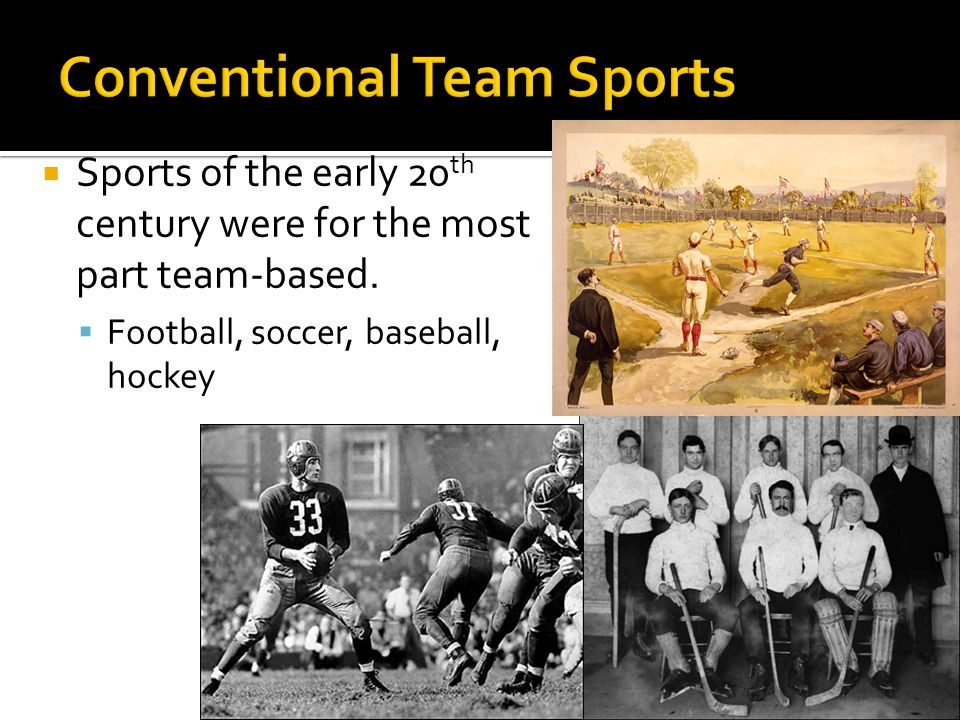The presentation slide titled "Conventional Team Sports" is designed with a black background and vibrant yellow text for the headline. Positioned on the left side, the slide features larger-than-body text that reads, "Sports of the early 20th century were, for the most part, team-based," followed by a smaller list of team sports: football, soccer, baseball, and hockey. On the right side, the slide showcases three historical images: at the top, an artistic color rendering of an old-time baseball game, distinguished by players in traditional uniforms; below left, a black-and-white photo depicting early 1920s football players donning minimal padding and leather helmets; and below right, another black-and-white photo of an early 1900s hockey team, with players posed with their sticks, wearing vintage athletic gear. The layout and content suggest a detailed examination of early 20th-century sports teams.